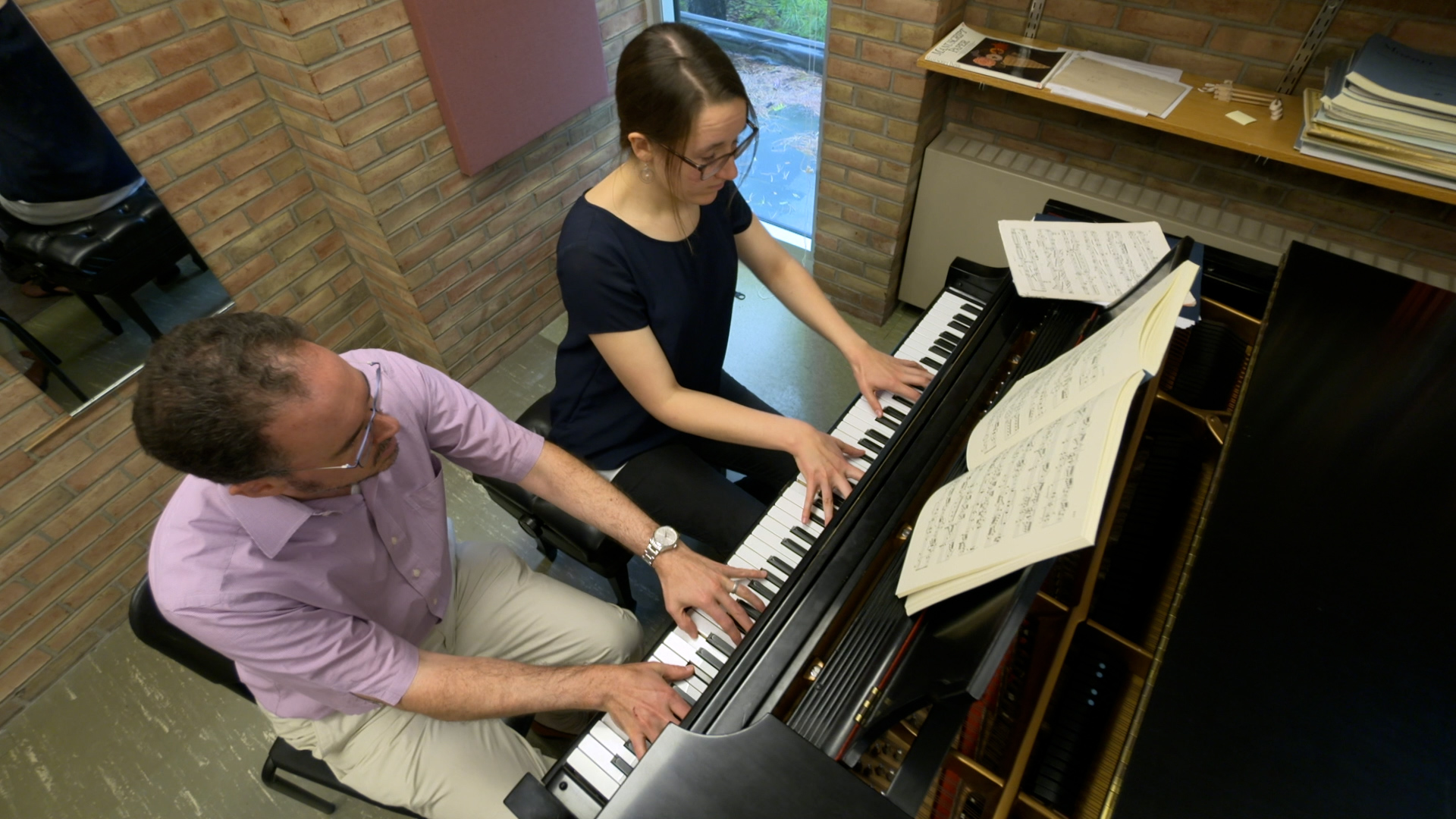In this image, two people are playing a black piano side-by-side, positioned in the right half of the frame and angled diagonally towards the top left corner. Captured from an overhead perspective, possibly from a balcony or higher floor, the scene reveals a crowded room with brick walls and linoleum tile flooring. A shelf filled with books and sheets of music is visible to the side, along with an open door leading outside.

The duo consists of a young woman and an older man, both wearing glasses. The woman, seated at the right end of the keyboard, has her hair pulled back, a blue shirt, gray pants, and earrings. The man, stationed at the left end, sports curly brown hair, a light lavender button-up shirt, beige slacks, and a silver watch on his wrist. He sits on a black chair, while she might be on a stool. Their fingers are poised on the keys, seemingly playing different notes while focusing on the open sheet music in front of them.

A mirror in the background reflects part of the piano, adding depth to the compact space. The detailed depiction of their clothing and the intimate setup suggests a deep concentration on their musical performance, hinting at either a teaching session or a practiced duet.